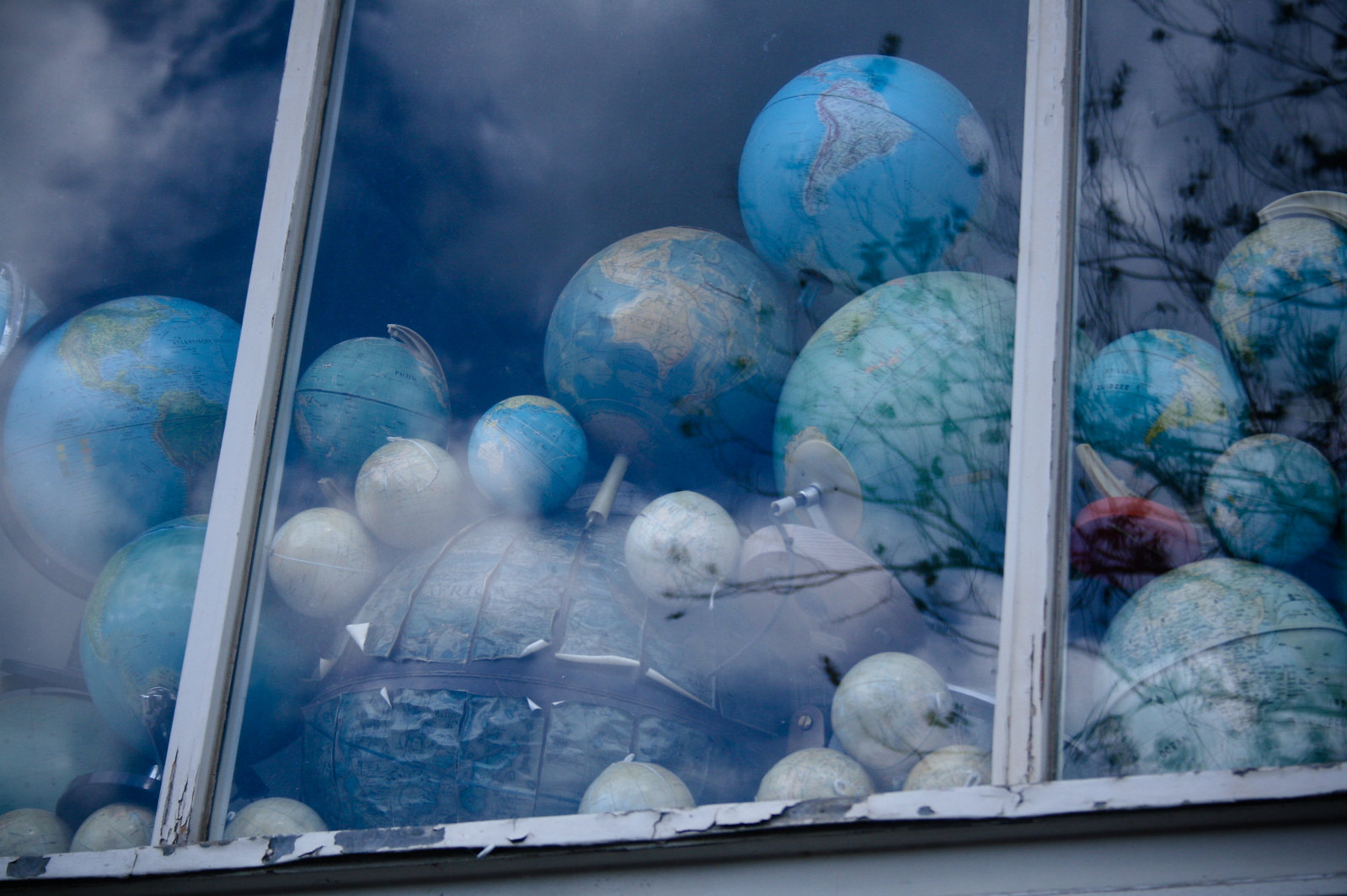This is an artistic close-up color photograph of a weathered window frame taken from the outside on an overcast day. The aging wooden frame is painted white, though the paint is peeling away noticeably towards the bottom. The window glass is divided into three panes, with the middle pane fully visible while the left and right panes are partially cut off by the edges of the image. Each pane is separated by white dividing bars, which mirror the window's worn and flaky condition.

Reflected in the glass, the cloudy sky and the sparse silhouette of tree branches add a melancholic touch. Within the dimly lit room beyond the glass, a fascinating collection of approximately 20 to 30 globes of various diameters are stacked. Most globes are in good condition, except for the largest one positioned at the bottom center, which appears to be in disrepair with flaking and wrinkled paper strips. Additionally, there are several white round objects resembling onions, and a large texturized case situated at the bottom center. A very light red unidentifiable object is also nestled among the globes. The predominant colors in the scene are white, light blue, shades of green, and gray, contributing to the overall muted and aged aesthetic.